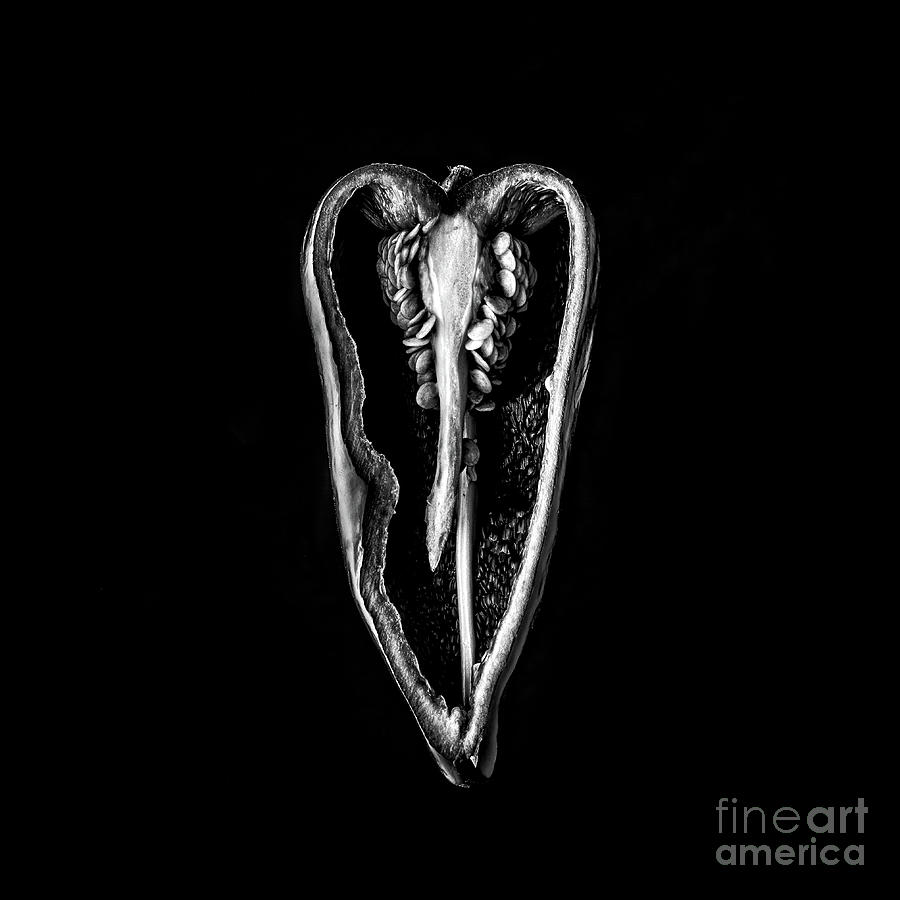The image features a striking composition against a black background, prominently marked with the watermark "Fine Art America" in gray at the bottom right corner. Dominating the center of the frame is a monochromatic representation that appears to be a cross-section of a pepper, sliced vertically. The shape resembles an elongated heart, and the high-contrast black-and-white coloration enhances its dramatic visual appeal. Inside the pepper, a distinctive long, lighter-colored structure descends from the top, evocative of a snake or tongue, flanked on either side by clusters of small, white seeds. The left side interior of the pepper is almost completely black, while the right side features black areas interrupted by white spots, creating a textured look. A line extends vertically through the center, adding to the complex, almost fossil-like appearance of the image.